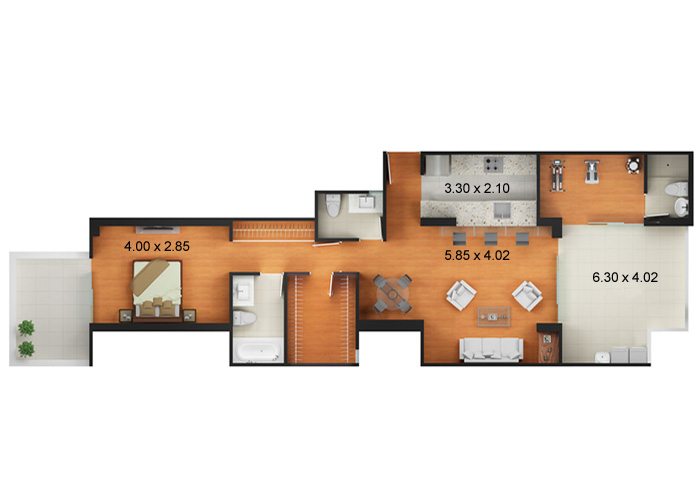This professionally rendered computer-generated floor plan illustrates a meticulously designed house layout. The plan features detailed measurements prominently in meters, ensuring clarity and precision.

**Left Side:**
- **Patio Area:** Situated on the left side, a slab adorned with potted bushes indicates an outdoor patio space, ideal for relaxation.
- **Garage:** Adjacent to the patio, a garage spans 6.30 meters by 4.02 meters, providing ample space for vehicle storage.

**Interior Spaces:**
- **Bedroom:** The first room next to the patio area is a cozy bedroom, furnished with a bed flanked by nightstands. This room measures 4.00 meters by 2.85 meters.
- **Bathroom and Hallway:** Proceeding down a narrow hallway, there is a bathroom equipped with a bathtub, toilet, and sink. Opposite this bathroom is a feature that might be either a staircase or a closet.
- **Walk-In Closet:** Farther along the hallway is a spacious walk-in closet, providing plentiful storage.
- **Additional Bathroom:** Continuing upward on the floor plan’s top portion is another bathroom, fitted with a toilet and sink.

**Central Living Space:**
- **Dining and Living Area:** An open area unfolds into a dining section with a table and chairs, seamlessly transitioning into a living room. This living space spans 5.85 meters by 4.02 meters and includes a bar area furnished with three bar stools and an ample counter.
- **Kitchen:** Adjacent to the bar area lies a compact kitchen, measuring 3.30 meters by 2.10 meters.

**Top Portion:**
- **Unspecified Room and Bathroom:** The top section of the floor plan reveals a brown-floored area that might be another bedroom or multifunctional space. This area includes three unidentified objects and leads to another bathroom equipped with a bathtub, toilet, and sink.

In summary, this detailed floor plan presents a well-thought-out layout combining outdoor and indoor spaces with essential amenities, ensuring comfort and convenience in a modern home setting.